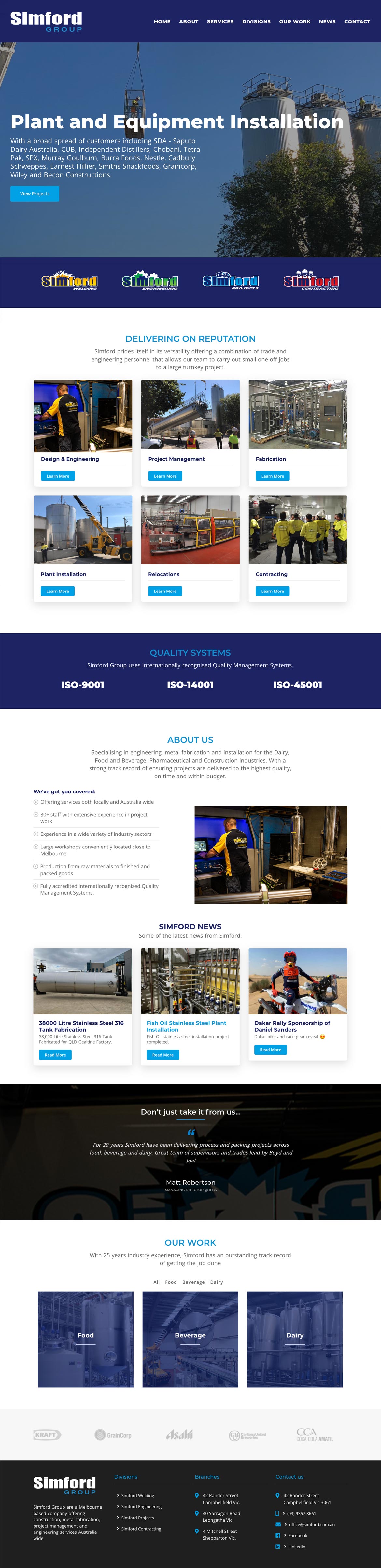The image features a largely white background with a prominent heading at the very top reading "Simford" in small, nearly indecipherable text. Directly beneath this, the text "Plant and Equipment Installation" is slightly more visible but still difficult to read. The central portion of the image showcases what appears to be three green silos surrounded by some trees. Below this main image are six small thumbnail images arranged in a row, each depicting varying details that are challenging to discern. Underneath these thumbnails is a dark blue rectangular box. Following this section, there are four more smaller thumbnails, set against another dark rectangular box, this time black in color. Lower down, there are three additional dark blue-colored thumbnails. At the very bottom of the image is another black rectangular box with "Simford" prominently displayed in large white letters. Throughout the image, there is a significant amount of text that remains largely unreadable, contributing to the overall cluttered and obscure appearance. Scattered within this scene are indistinct figures that suggest the presence of people, though their details are lost in the blurriness of the image.